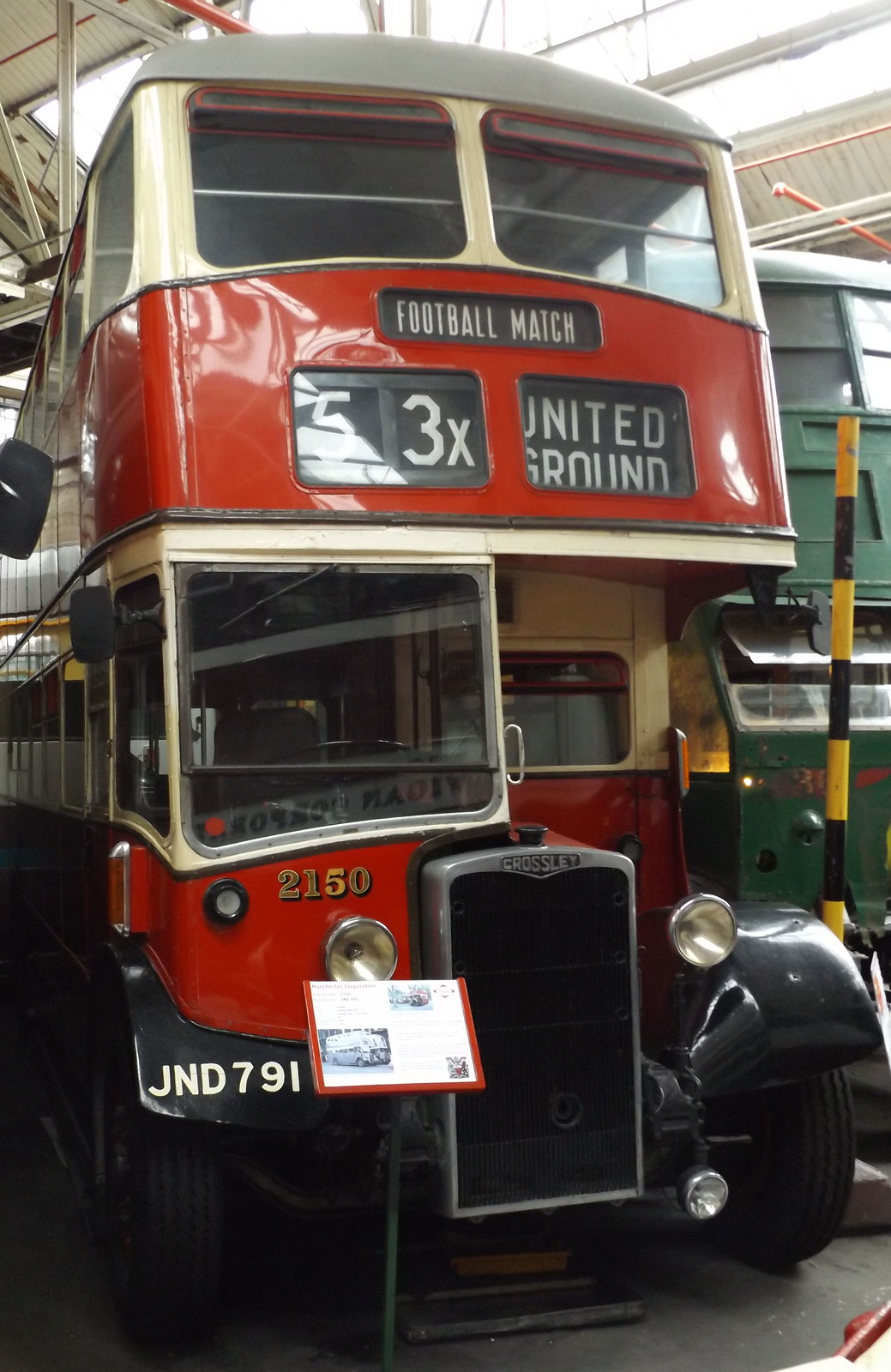This color photograph, in a portrait orientation, captures the front end of an old-fashioned double-decker bus, which is part of an indoor exhibit of antique buses. The bus exhibits a vintage design with a shiny metallic red body and white trim around the windows. The top deck features black screens with white text reading "Football Match" and "53X United Ground". The lower section displays a black and white reader section, along with an old-fashioned vertical rectangular radiator grille framed in light gray. Positioned at the lower left fender is the license plate "JND 791", next to a white placard mounted on a stand, containing illustrations and information about the bus, suggesting a museum setting. The image also shows part of another bus in green to the right, further emphasizing the exhibition environment. The detailed realism of the photograph highlights the intricate design and historic charm of the bus.